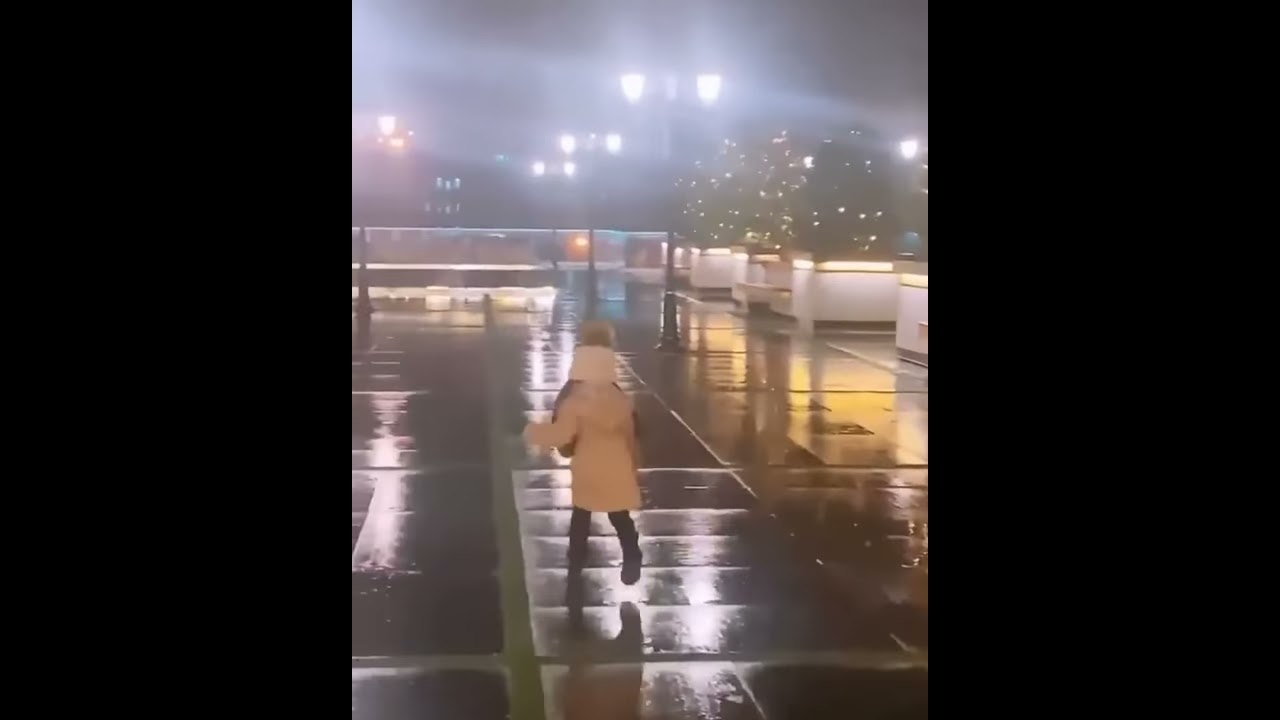The image captures a small figure, potentially a child or a petite woman, running across a wet, concrete courtyard at night. The scene is illuminated by multiple street lights, which cast a reflective glow on the puddled pavement. The runner is clad in dark pants, sturdy boots, and a large tan coat that reaches her knees, with her head covered by either a hood or a large hat. Her right foot is lifted mid-stride, emphasizing her rapid motion. The courtyard is bordered on the right by white walls featuring brown sections, and neatly trimmed hedges set in pillars with festive lights. A five-foot-tall concrete wall adorned with additional lights and trees forms the background, beyond which illuminated buildings stand out against the night sky. Despite the overcast weather, indicated by the diffuse aura of light through the rain, the scene feels vibrant yet isolated, with most peripheral areas shrouded in darkness.